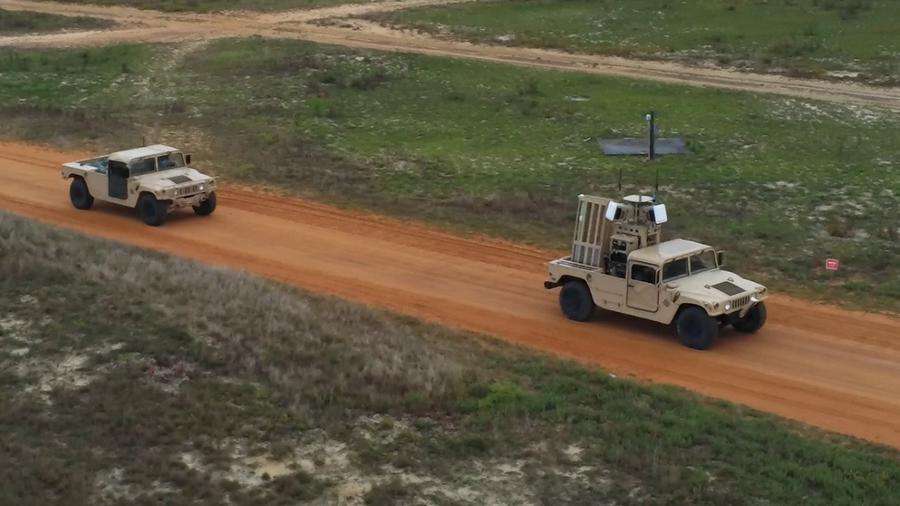The image appears to be a drone photograph, capturing two cream-colored Humvee-style military vehicles traveling on a brown dirt road in a remote and sparsely grassed area. The landscape features green grass on either side of the road, intersected by an additional grayish-brown dirt path. The vehicle on the left seems to contain some wires or electronics, while the one on the right holds a large device, possibly for weather monitoring, wind analysis, or radar detection. The right vehicle is passing by a red, unreadable sign. The scene, set under a dreary sky, hints at a military installation or research area, with a black box visible in the grass, potentially used for parking or charging military equipment. The environment suggests an arid climate, possibly Mediterranean.